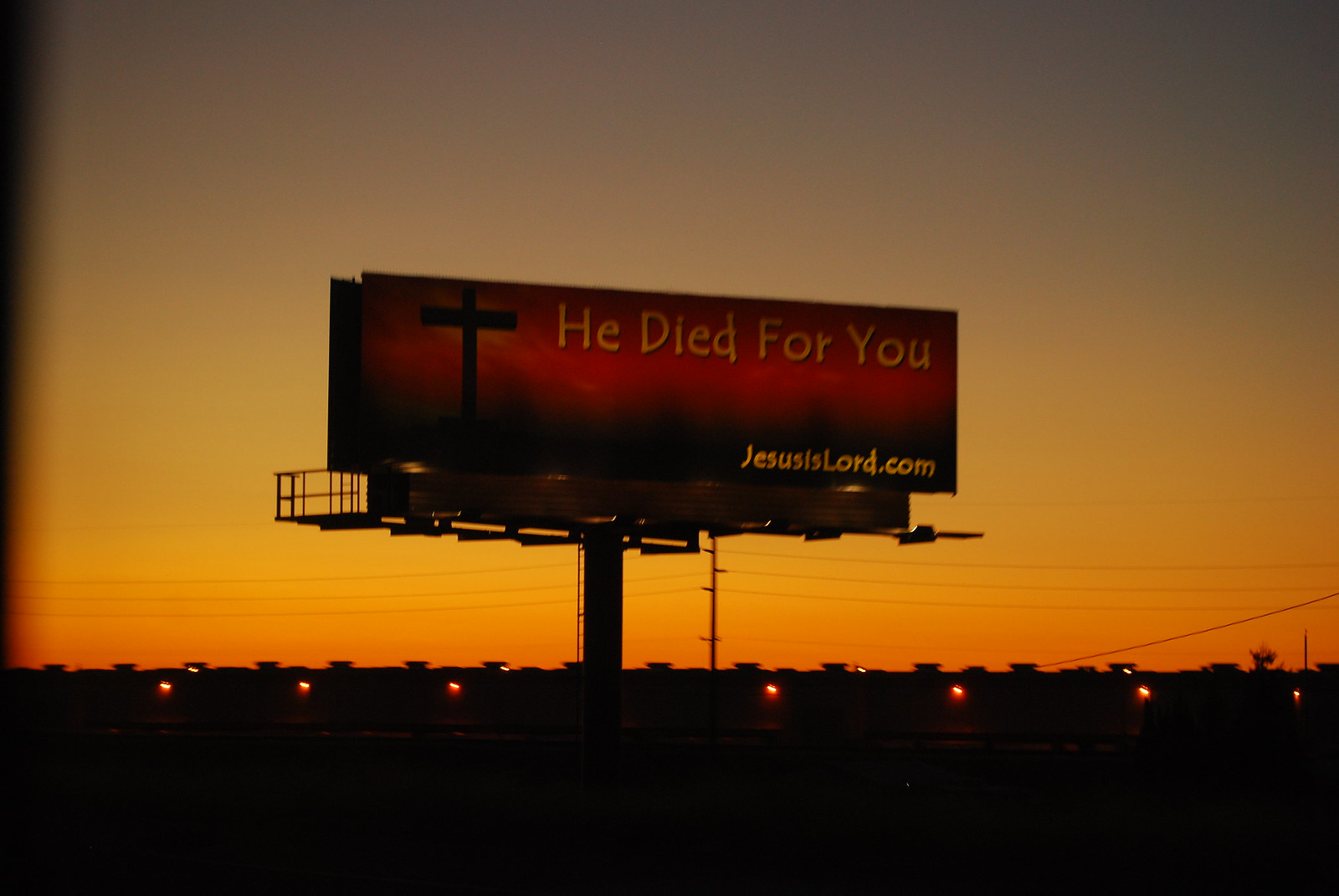This photograph captures a striking billboard during sunset. The sky behind the billboard glows in a gradient of orange, yellow, and peach hues, creating a dramatic backdrop. The billboard itself is predominantly red, transitioning to black at the bottom. Emblazoned at the top in bold yellow letters are the words "He died for you," while the bottom right corner displays "JesusIsLord.com" in the same yellow text. On the left side of the billboard, a large black cross stands out. The billboard is illuminated by lights, casting a distinct glow that contrasts with the darkening skyline and silhouetted structures in the distance, which resemble castle walls. Below the billboard, the scene includes evenly spaced lights and a faint outline of houses, surrounded by a grassy area and a fence, with power lines and telephone poles visible in the background. This photograph, rich in detail and color, emphasizes the juxtaposition of the religious message with the serene yet vibrant sunset.